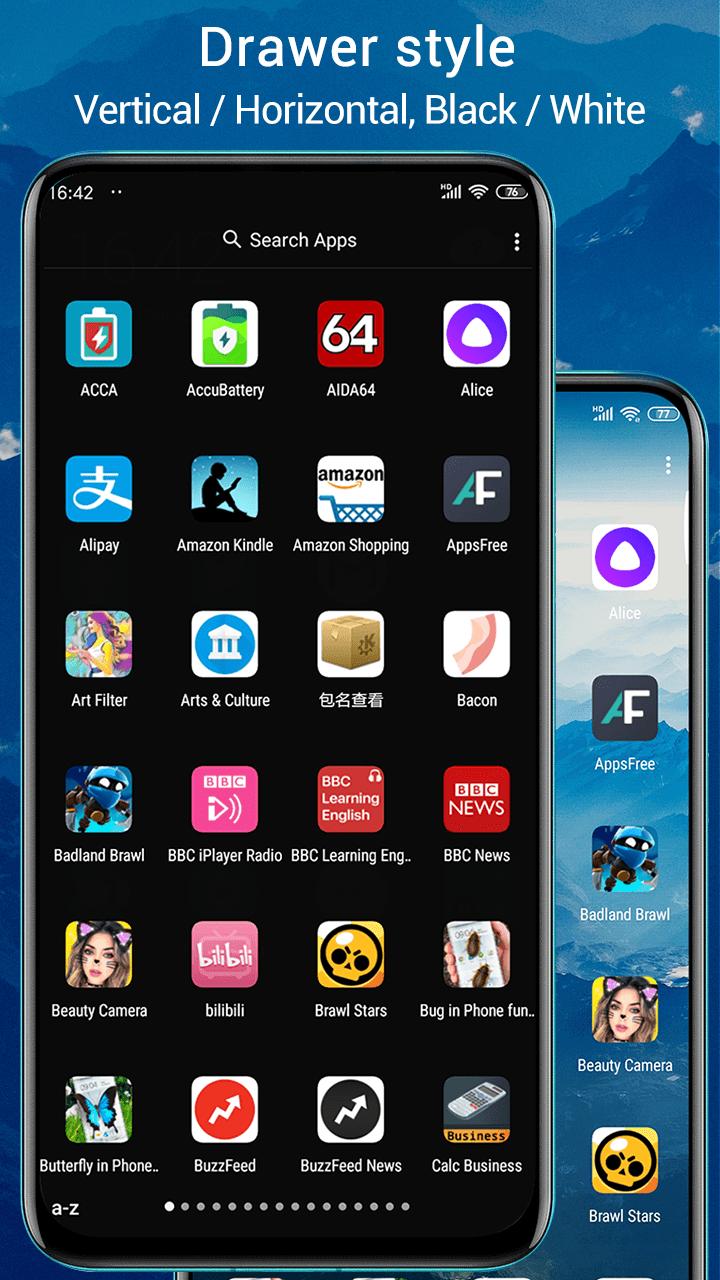The image showcases a website featuring a distinct blue-tinted mountain backdrop. At the top of the webpage, white text displays the phrases "drawer style," "vertical slash," "horizontal comma," and "black slash white." Below this, a screenshot of a phone screen is prominently displayed. The phone screen features a search bar labeled "Search apps" and displays 24 apps set against a black background. Visible app icons include ACCA, AccuBattery, Alice, BBC Player Radio, Arts & Culture, BuzzFeed News, Beauty Camera, Art Filter, and All Play. 

In the background of the image, there is another partial screenshot of a phone screen with a gradient background consisting of light blue, dark blue, and medium blue shades. This secondary screenshot highlights five available apps: Brawl Stars, Beauty Camera, Badland Brawl, Apps Free, and Alice.